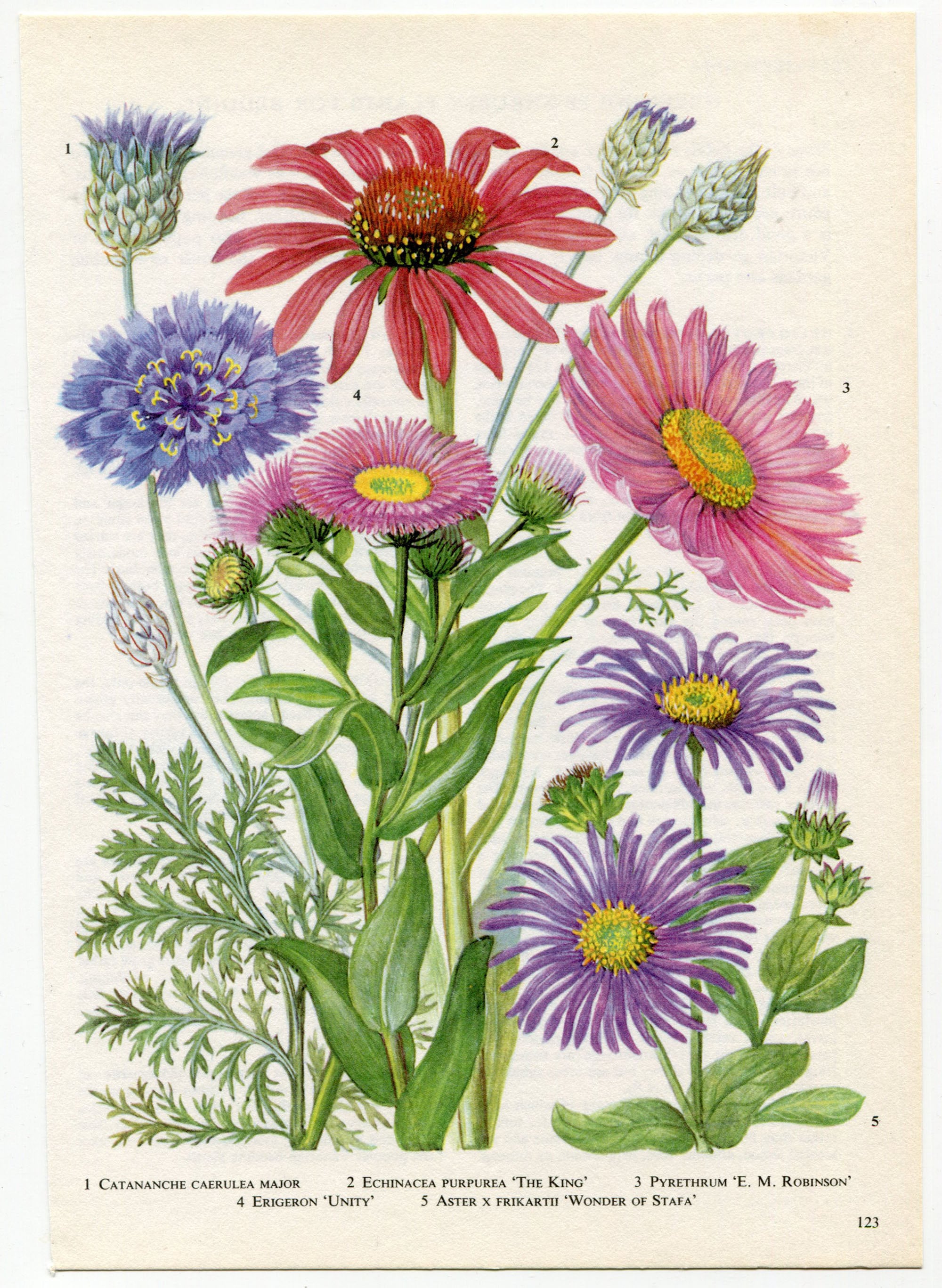This illustration, likely from an aged book or magazine, depicts a detailed, color-plate of various flowers, arranged against a beige background indicative of old paper. The flowers are diverse in shape and color, showcasing red, pink, purple, and blue hues, with each specimen meticulously labeled with a number corresponding to its Latin scientific name listed at the bottom in a small, uppercase font. Notably, the blue carnation stands out among the collection. The central top flower features striking red petals encircling a black center with yellow dots and delicate red fibers, flanked by purplish blooms. Flowers with branching, daisy-like petals and yellow centers are prevalent, some still in bud form. The legend identifies the flowers with names like 'Catananche cerulea major,' 'Echinacea purpurea,' 'Pyrethrum E.M. Robinson,' 'Erigeron unity,' and 'Aster x fricartii Wonder of Staffa.' There appear to be five main flowers pictured, each meticulously rendered to capture their unique botanical characteristics.